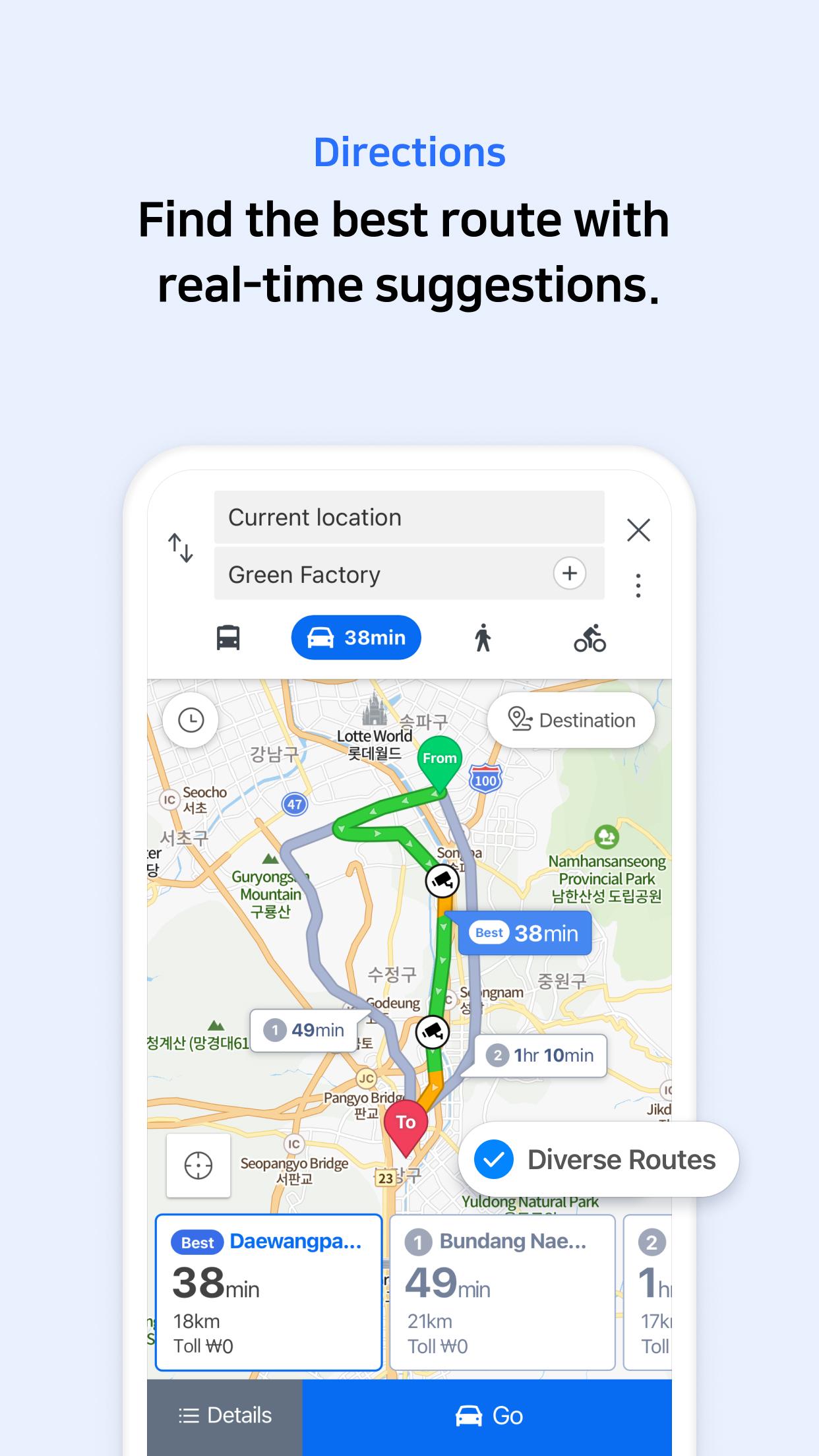**Detailed Caption for the Advertisement Image:**

The advertisement prominently showcases a navigation application, likely Apple Maps, based on its design elements. The focal point of the graphic is a section titled "Directions: Find the Best Route with Real-Time Suggestions." The map display highlights a route from the user's current location to a destination referred to as "Green Factory." Two route options are illustrated: one is the "best route," spanning 18 kilometers and taking approximately 38 minutes, while the alternative route is 21 kilometers and requires 49 minutes to traverse. Some routes appear to include toll roads. 

The map insert is notable for its inclusion of Asian characters, suggesting the location could be in an Asian country, potentially China. Specific landmarks such as “Pangyo Bridge” and “Yuledong National Park” are marked on the map. Once the user decides on their preferred route, they can initiate real-time navigation by pressing a prominent blue "Go" button at the bottom of the screen. This seamless integration aims to enhance the user experience by providing efficient and accurate navigation options.